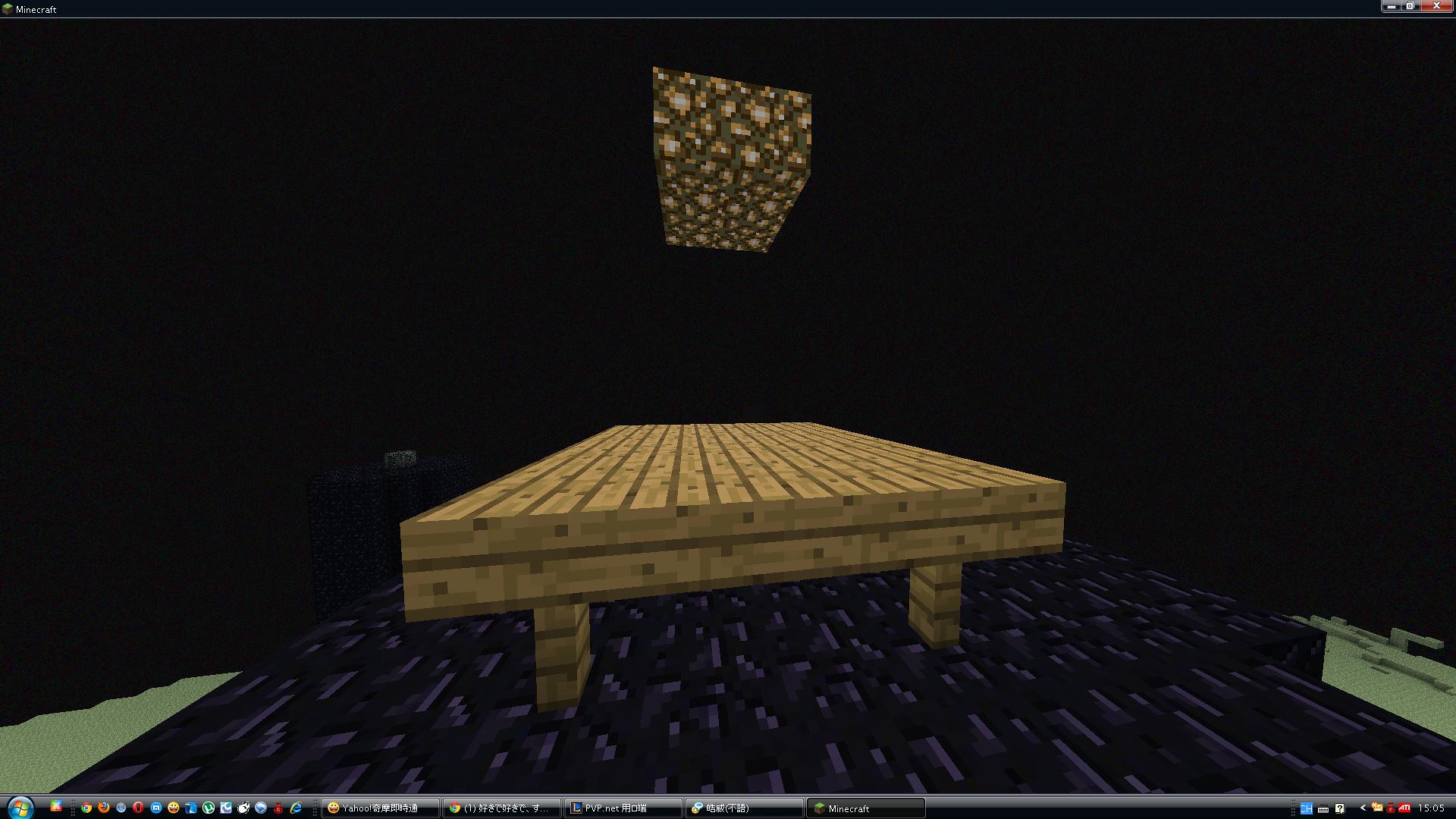Screenshot from Minecraft in windowed mode on a Windows 8 desktop. The window's title bar shows "Minecraft," characteristic of the old Windows 8 style, with a black taskbar at the bottom and icons arranged on the left, including the Windows icon for the Start menu. The game view captures a wooden deck standing above obsidian blocks, surrounded by an area dominated by darkness. A glowstone block is visible, attempting to illuminate the scene. The environment suggests the player is in the Nether realm, known for its low-light conditions and ominous shadows. The player appears to be in the process of brightening and constructing within this challenging, dark territory.